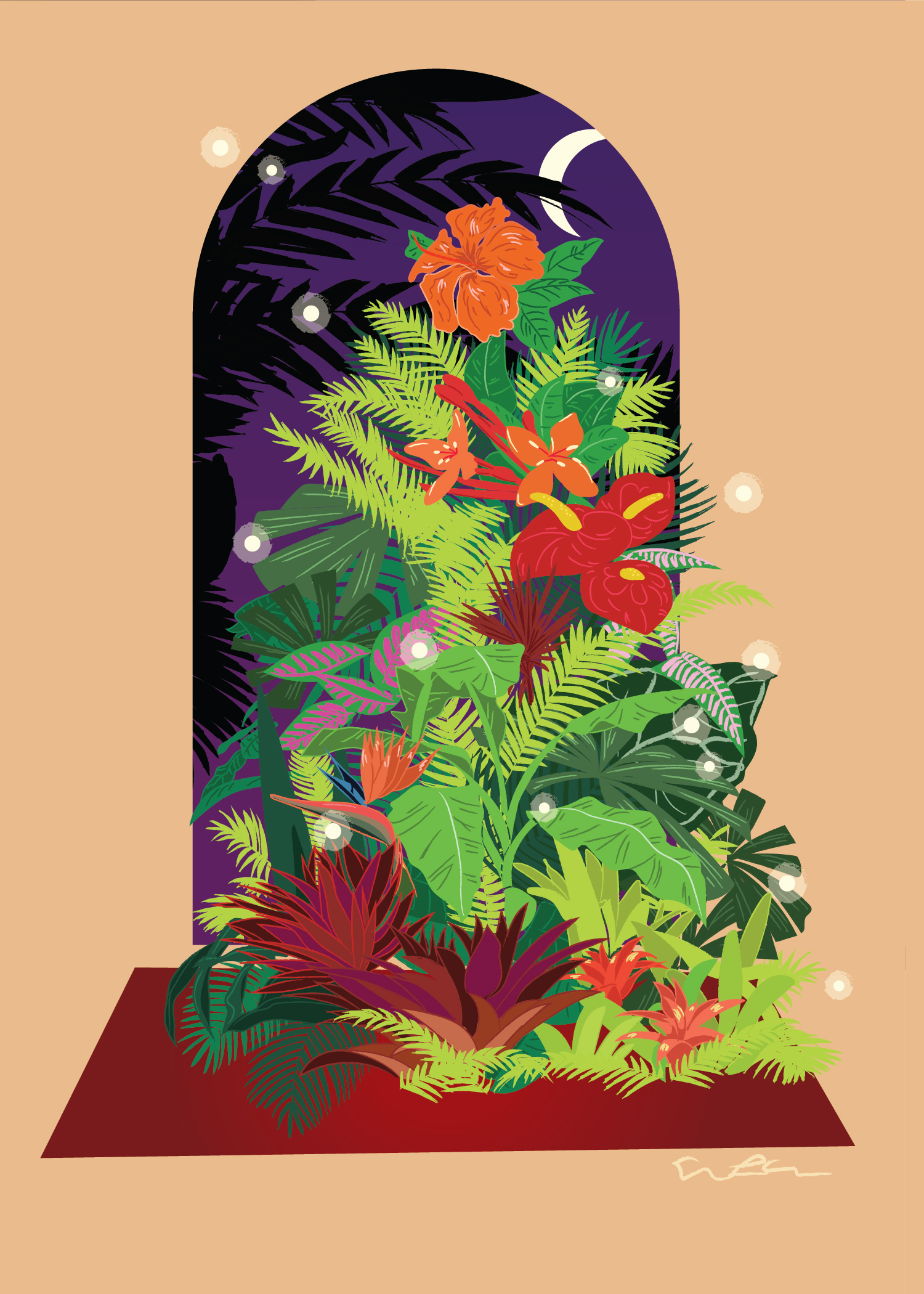In the image, we see an arched passageway that opens onto a serene nightscape. The sky is a rich purple, adorned by a delicate crescent moon positioned in the upper right, and framed by the dark silhouettes of palm fronds and other tree branches with leaves. Just inside the arch, the wall is painted a warm peach color, adding to the cozy atmosphere.

In front of the archway, a red mat lies on the floor, anchored towards the bottom of the image. On this mat, there is an impressive arrangement of plants and flowers, stacked in a tier resembling a Christmas tree. This verdant display features a variety of leaves in light, medium, dark, and even darker shades of green. Amongst the foliage, vibrant flowers in hues of orange, red, purple, and dark rose create a colorful mosaic. Notable blooms include an orange hibiscus and a distinctive red flower with a yellow stem. 

The scene is punctuated by mysterious white circles with lighter halos around them, floating ethereally throughout the room, adding a magical, almost whimsical touch to the tranquil setting.